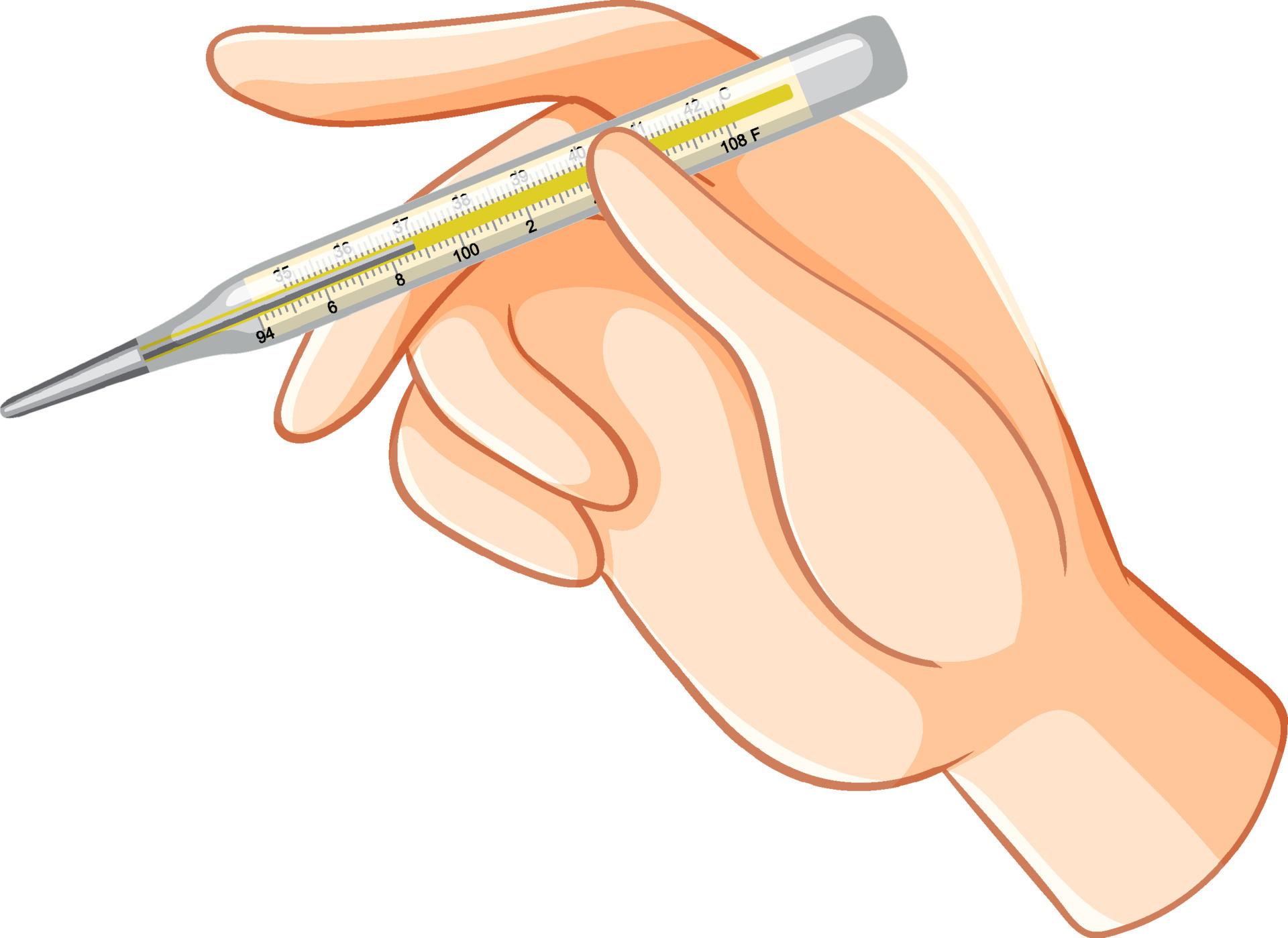The image is a detailed clip art illustration of a right hand holding a mercury thermometer. The hand, which appears to be male, is depicted with a pale tan shading and a brown outline, filled with various shades of pink, ranging from light to medium tones, and a slightly darker peachy flesh color. The hand holds the thermometer delicately between the thumb and pointer finger, similar to how one would hold a pen. The thermometer is metallic silver with reflective white highlights, and it is held diagonally with the tip pointing downward to the left. The temperature displayed ranges from 35 to 42 degrees Celsius (94 to 108 degrees Fahrenheit), showing a reading of approximately 37 degrees Celsius or 98.6 degrees Fahrenheit, indicating a normal body temperature.